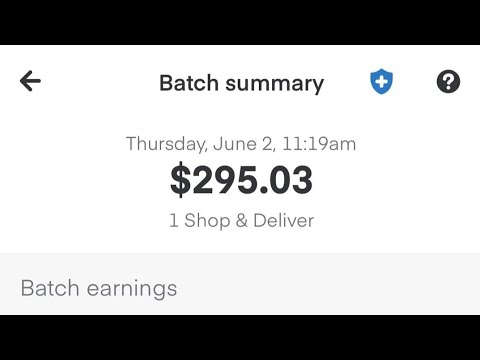A cropped screenshot displays the end-of-day sales summary for a gig worker. The top and bottom of the image feature horizontal black bars, indicating the areas where the image has been cropped. Dominating the center of the screenshot, the heading "Batch Summary" is displayed prominently in large black font. To the left of this heading, there is a back arrow icon, allowing navigation to the main screen. On the right side, a blue shield icon with a white cross is visible, followed by a question mark icon.

Centered within the image, the date "Thursday, June 2nd, 11:19 a.m." is clearly shown. Directly below the date, a substantial amount of "$295.03" is presented in large black letters. Underneath this amount, the phrase "1 Shop and Deliver" is centered in black font.

Towards the bottom of the screenshot, a gray rectangular section labeled "Batch Earnings" appears on the top left in large gray letters, marking the lower portion of the display.